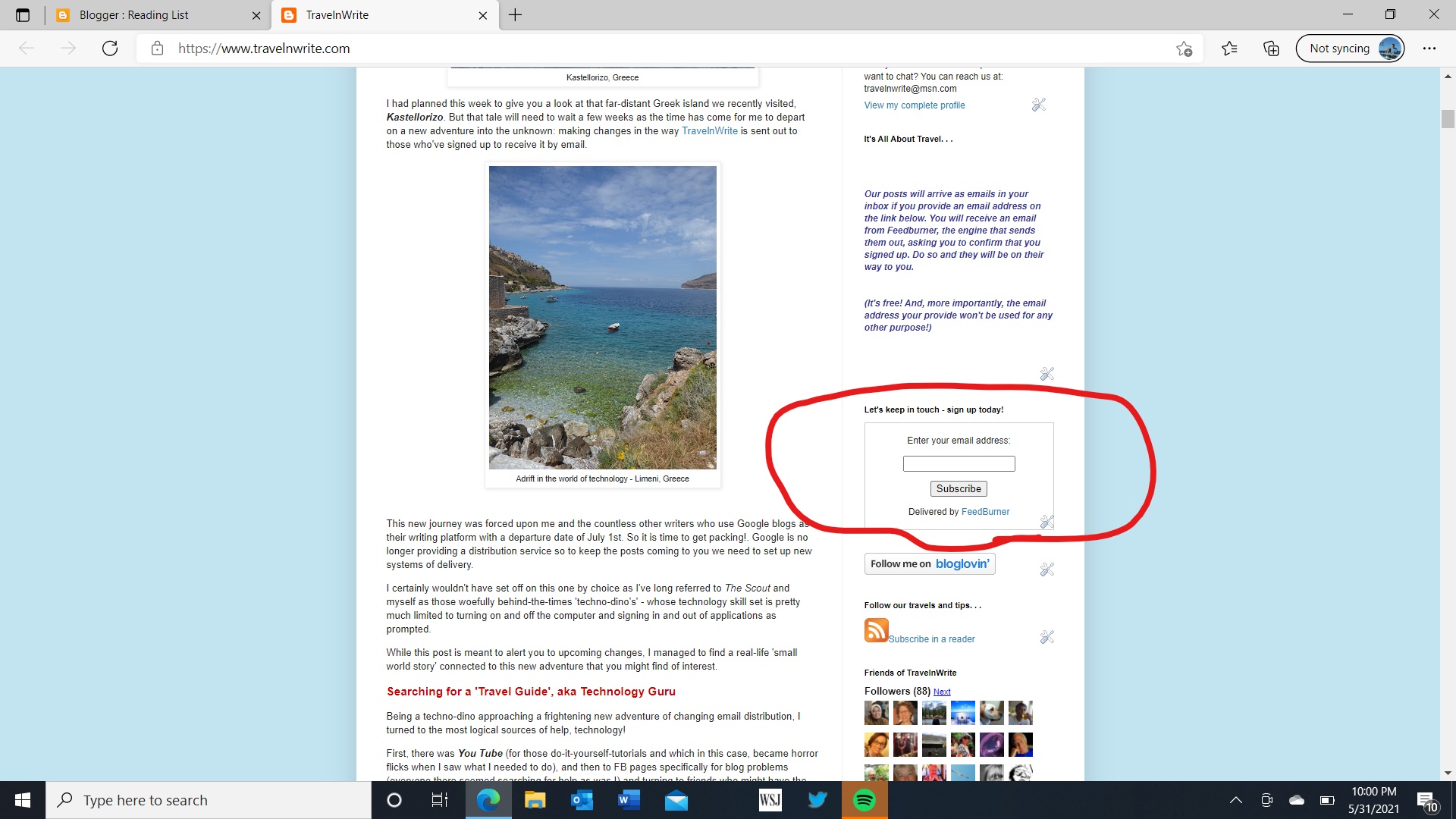The image captures a screenshot from a webpage, likely from the website travelandwrite.com, which can be viewed on both mobile devices and desktop computers, owing to its size and layout. At the top of the page, there is an announcement that reads: "I had planned this week to give you a look at that far distant Greek island we recently visited, Castel Rezo, but that tale will need to wait a few weeks as the time has come for me to depart on a new adventure to the unknown, making changes in the way Travel and Write is sent out to those who've signed up to receive it by email."

Below the announcement is an image titled "Adrift in the World of Technology, Limeni, Greece," depicting a stunning water scene flanked by rock, grass, and stone formations on both sides under a clear blue sky. The author continues, discussing the quest for a technology guide or guru to assist with these changes, mentioning the exploration of YouTube and DIY tutorials.

Towards the bottom of the page, there is a call-to-action for visitors to stay connected by signing up for email updates. This section includes a field to enter an email address and a "Subscribe" button. The area has been highlighted with a red Sharpie circle, drawing attention to the sign-up prompt in the middle of the page.